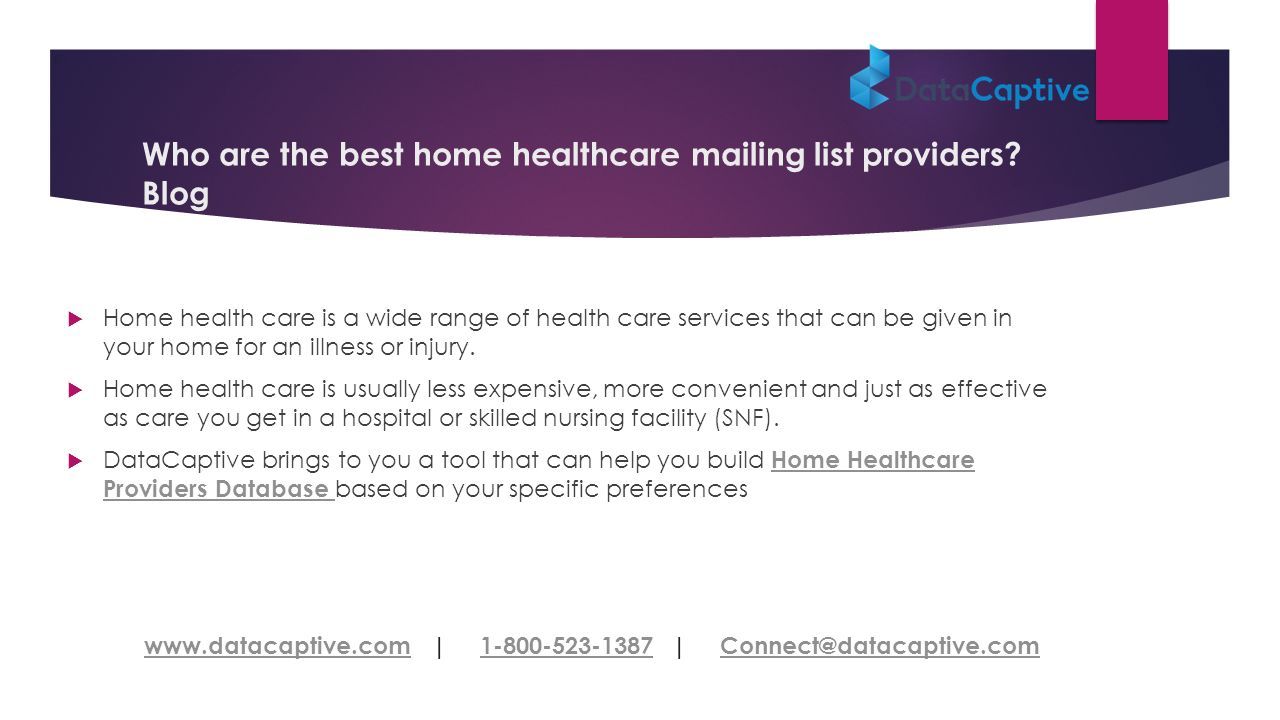The image appears to be a polished advertisement for Data Captive, presented in a color format. The composition features a sophisticated, sleek design, with a banner prominently displayed at the top. The banner has a curved, modern aesthetic in a purplish hue, with bold white lettering asking, "Who are the best home health care mailing list providers?" suggesting this is blog content.

The logo of Data Captive, positioned prominently, is an almost-completed blue cube, with one side artfully flipped upward, giving it a dynamic and modern appearance.

Immediately below the heading, the content is organized into three bullet points, each providing valuable information about the nature and benefits of home health care. 

1. **Home health care is a wide range of health care services that can be given in your home for an illness or injury.**
2. **Home health care is usually less expensive, more convenient, and just as effective as care you could get in a hospital or skilled nursing facility (SNF).**
3. **Data Captive brings to you a tool that can help you build a home health care providers database based on your specific preferences.** *(The phrase "home health care provider database" is hyperlinked for ease of access.)*

At the bottom of the image, contact information is provided, including a phone number and an email address for further inquiries, ensuring easy access to more information. Overall, the advertisement exudes professionalism and serves as an informative resource for those interested in home health care services and Data Captive's offerings.